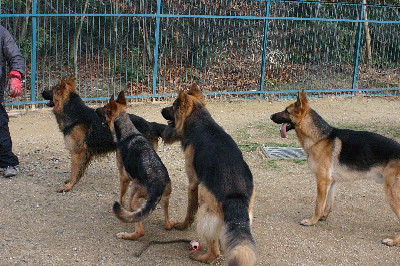In this detailed photograph, four large dogs, predominantly German Shepherds with characteristic black and tan markings, are intently focused on a person partially visible on the far left of the image. The person, presumably a trainer, is clad in a bulky blue jacket, matching pants, and a pronounced red glove on their left hand, suggesting a training or command scenario. These dogs, two of which have longer fur, stand on a gravelly, dirt-strewn ground. The rightmost dog has its tongue sticking out. The scene is enclosed by a blue fence, with green foliage visible beyond it. There's a vent visible in the middle of the ground, adding to the enclosed training environment's detail. All dogs are looking attentively towards the trainer, indicating their high level of interest in the red-gloved hand.